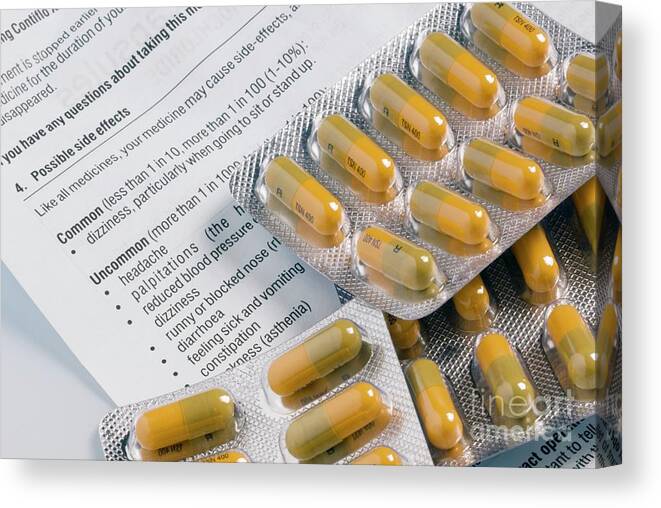The close-up photograph features three packages of capsules with a Fine Art America watermark in the lower right-hand corner. Each capsule is half dark green and half yellow, and they are contained within bubble packs of 10. The left portion of the image is largely occupied by drug information paperwork that elaborates on the medication's potential side effects, detailing both common and uncommon reactions. Among the common side effects, it mentions dizziness, particularly when standing up or sitting down. Uncommon side effects listed include headache, palpitations, reduced blood pressure, runny or blocked nose, diarrhea, nausea and vomiting, and constipation. The text further notes that side effects can occur with any medication. Some parts of the text are obscured by the pill packaging, but the visible details provide a thorough overview of the drug's side effect profile.